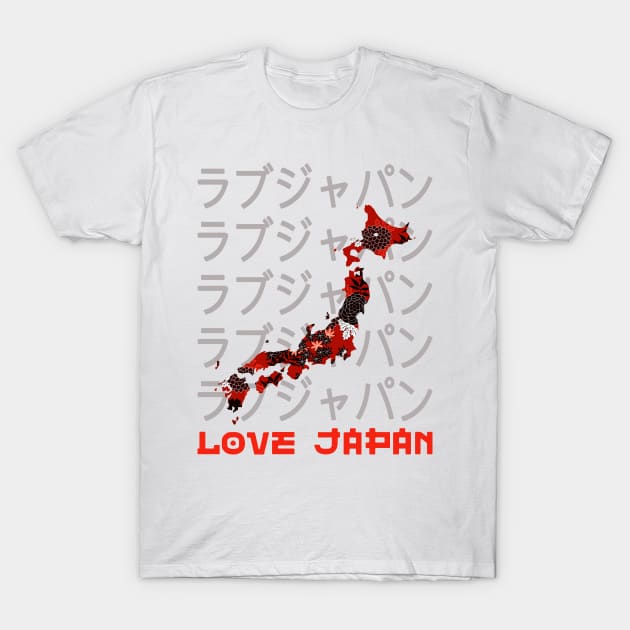This image features a regular, short-sleeved white t-shirt with a crew neck collar, displayed on a matching white background. The standout design element on this t-shirt consists of repeated Japanese lettering arranged in five rows across the front. Superimposed over these gray Japanese characters is a stylized representation of the map of Japan, depicted in varying floral patterns. Within this map, some islands are highlighted in red and others in black, with two gold stars marking specific locations, possibly referencing significant cities like Hiroshima and Osaka. Below the map, the phrase "Love Japan" is prominently displayed in bold red text, emphasizing the cultural and artistic theme of the garment.